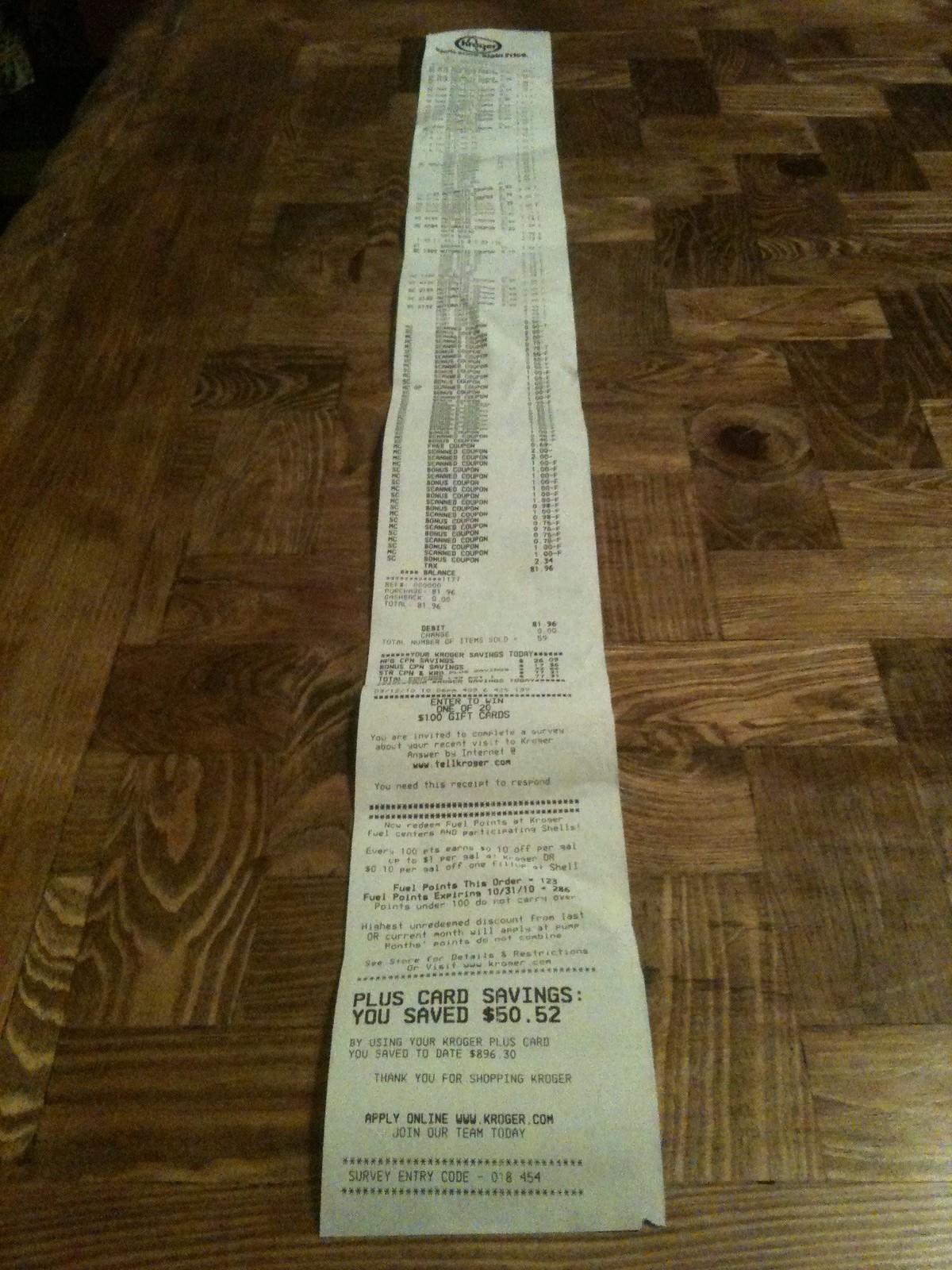This color photograph, taken in artificial light, captures an impressively long receipt from a Kroger store, stretching vertically from the very top of the image to the very middle bottom. The white, crinkled receipt contrasts with the black text detailing numerous purchased items, which include a notably regular pattern of repeated purchases in one section. The bottom of the receipt proudly states "Plus card savings: You saved $50.32" in bold text. Additionally, the receipt ends with the prompt to apply online at www.kroger.com. The entire receipt is laid out on a brown, laminated wooden table that features subtle carvings and a yellowish tint due to the lighting, adding warmth to the scene. The focal point is sharp with gradual blurring toward the top, emphasizing the impressive length of the receipt.